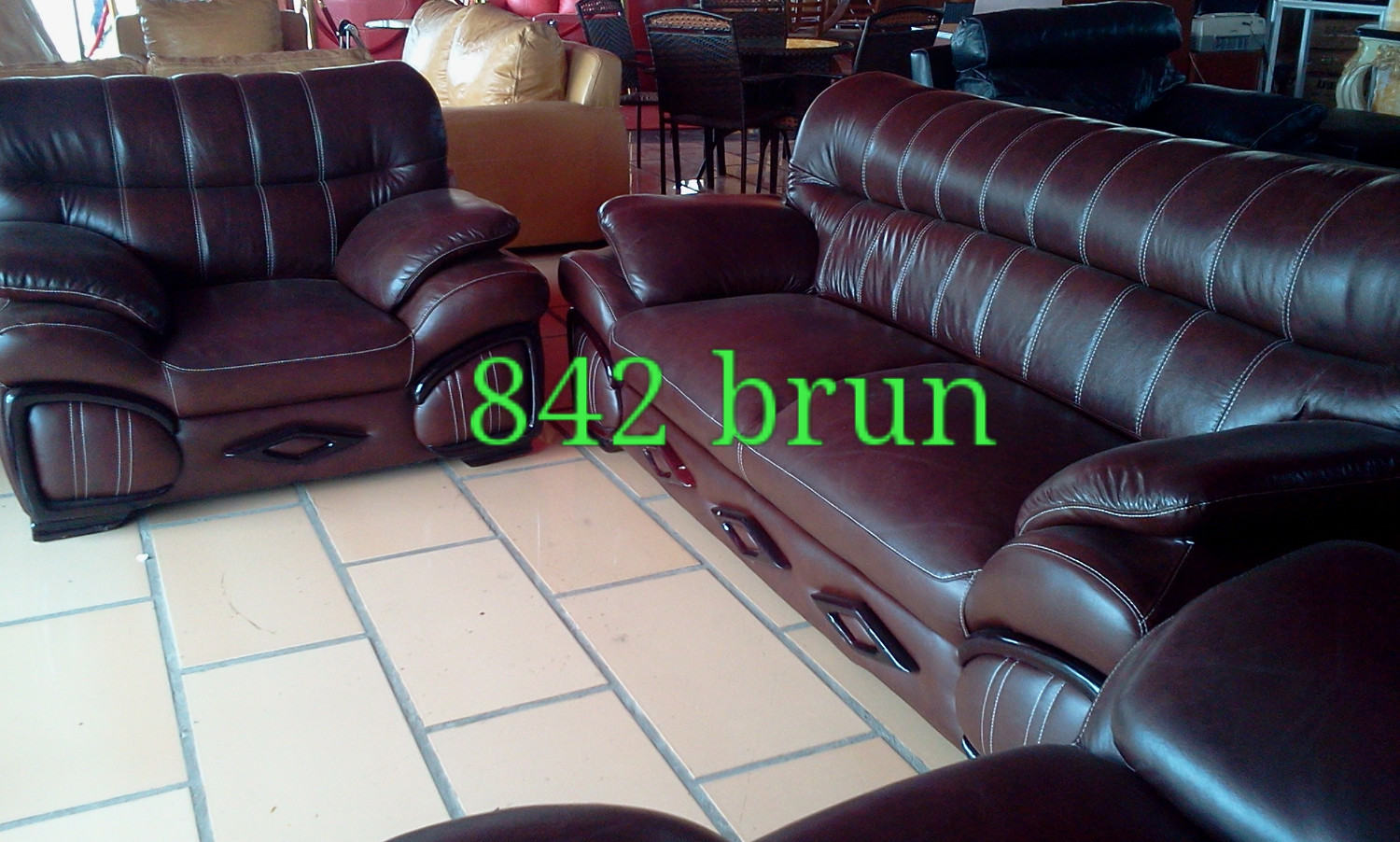The image depicts a detailed interior of a furniture store. The foreground showcases a burgundy leather furniture set consisting of a plush, heavily cushioned single-seat chair with an embossed design on the footrest area and a coordinating long sofa with white stitching on the back cushions, capable of seating three people. Both pieces rest on large, beige tiled flooring. Adjacent to these main furniture highlights, partially cut off, is another piece of matching furniture. In the background, various other furniture sets are visible, including another beige sofa set, a dining table with four chairs, and possibly additional couches and decor like a large vase. Bright green text reading "842 Brun" is prominently displayed across the center of the image, likely indicating a color designation for the sofas. Clear windows and faint glimpses of people walking past add dimension and context to the store’s layout.